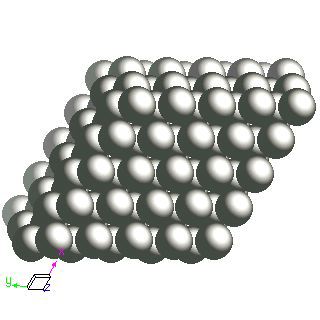The black-and-white image depicts a complex arrangement of interconnected spheres, forming a multi-layered structure. Positioned centrally, the spheres are arrayed in a grid with horizontal rows and vertical columns, presenting a three-dimensional effect. The structure comprises five horizontal rows, each with seven vertical layers, creating a rectangular prism-like shape resembling a scientific model. In the bottom left corner, a small diagram features two white boxes with black trim, alongside a numeral or letter, possibly a "2" or "Z". Adjacent to this, a bright green arrow points left, marked with a "Y", and a pink arrow directs upwards towards the sphere arrangement. Additionally, purple arrows extend diagonally upwards from a parallelogram shape. The spheres exhibit shading, with darker tones at the top, giving a shadowed appearance as they recede into the background.